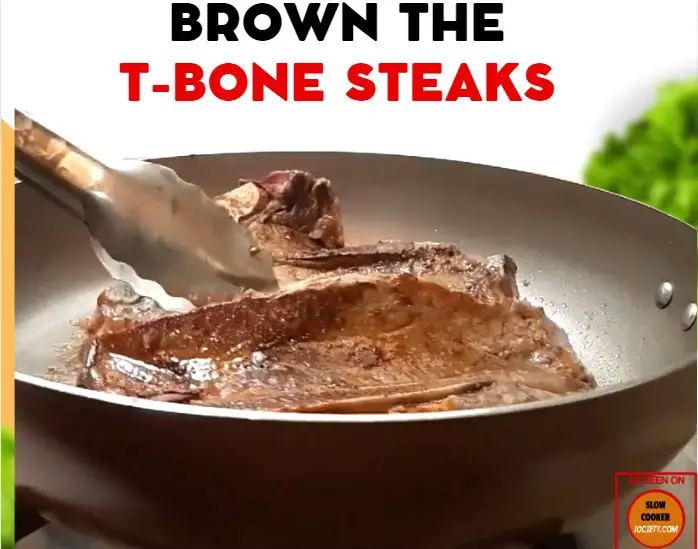The image showcases a close-up of a searing T-bone steak in a non-stick cooking pan, likely made of bronze or brown on the outside and silver on the inside. The steak, rich brown in color, rests in a sauce or marinade. Silver tongs are shown grasping the steak, possibly to flip it. The scene is detailed with additional elements like a plain white background, some green lettuce in the upper right corner, and a tan cutting board. Text at the top of the image, with "Brown The" in black and "T-Bone Steaks" in red, indicates the cooking process. In the bottom right corner, a red box contains the text "as seen on slowcookersociety.com," though the URL is somewhat blurred. The detailed colors present in the image are black, white, red, green, brown, gray, and orange. The style suggests a format suitable for a website or a TV cooking show.